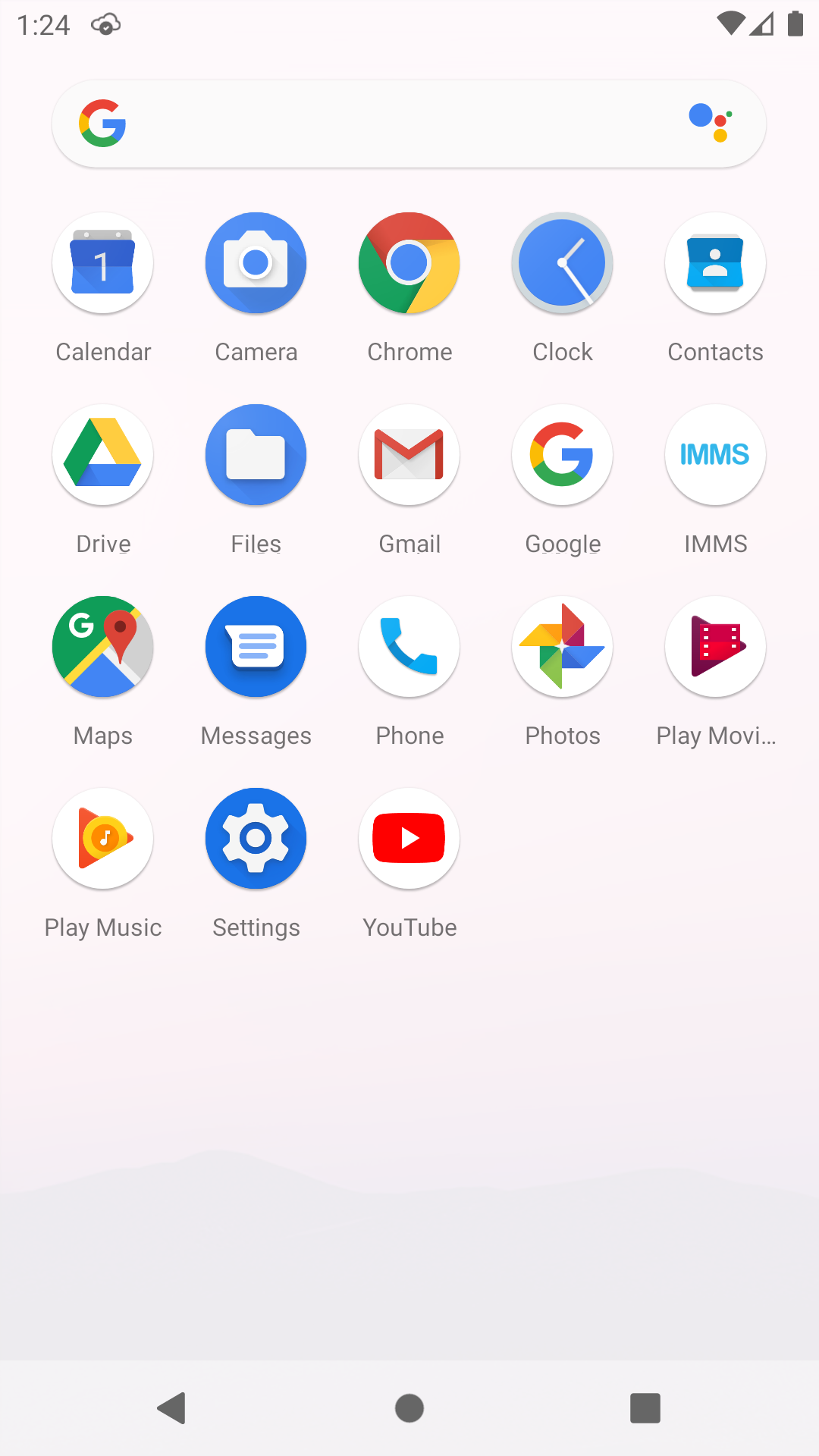The image portrays a smartphone interface featuring a home screen with various app icons. The apps displayed include Calendar (number 124), Camera, Chrome, Clock, Contacts, Google Drive, Files, Gmail, Google Search, IMMS (with all letters in capital), Maps, Messages, Phone, Photos, Play Movies (partially displayed as 'MOVI...'), Play Music, Settings, and YouTube. At the bottom of the screen, there are navigation icons: an arrow pointing left, a circle, and a square. Additionally, the top portion of the screen showcases a search bar marked by a Google logo rendered in red, yellow, green, and blue, accompanied by a multi-colored circle (blue, red, and yellow) with a central green dot to the right of the search bar.